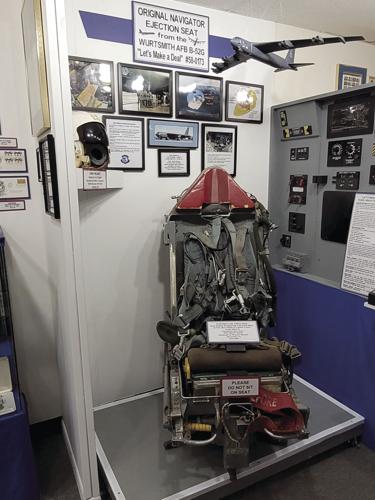This highly detailed photorealistic image depicts a meticulously curated exhibit within a historical Air Force museum, prominently featuring the original navigator ejection seat from the Wurtsmith AFB B-52G, labeled with the sign "Let's Make a Deal, 5B-0173." The seat itself, adorned with brown fabric, various buckles, straps, and what appears to be an integrated vest, is mounted on a pedestal with a clear sign instructing, "Please do not sit on seat. It is on display." Surrounding the seat, the exhibit includes an array of framed photographs and informational plaques detailing the airplane's history and the ejection seat's role within it. To the right, a wall-mounted array of cockpit instruments, buttons, and levers offers a glimpse into the avionics used to operate the aircraft. Suspended from the ceiling is a precise balsa wood model of the B-52G, adding depth and context to the exhibit. Additionally, a shelf on the left holds a helmet, presumably used by the navigator who once occupied the ejection seat, adding a personal touch to the display. The leftmost section of the image hints at another display, although its contents remain unclear.